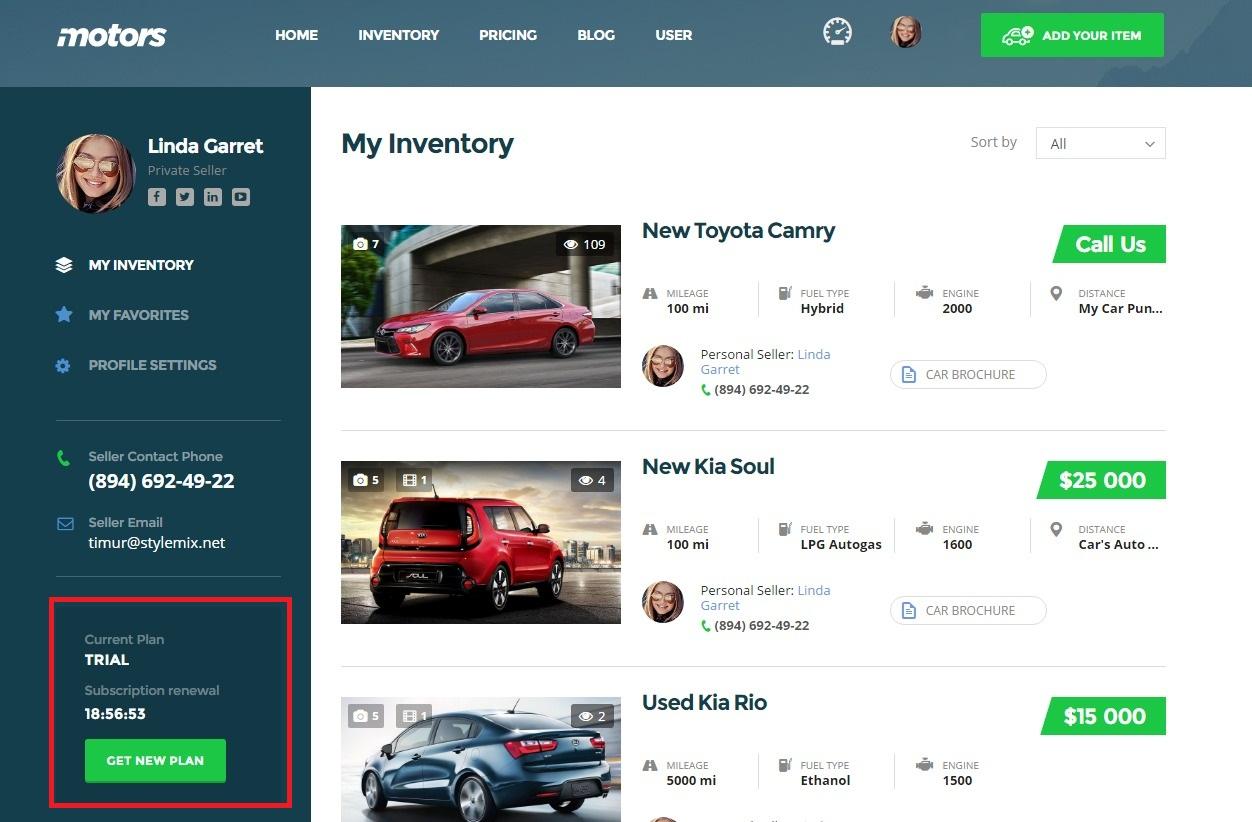The image is a detailed screenshot of a website with a light teal background at the top. The header features a white logo with the word "motors," all in lowercase letters. Next to the logo, there are navigation links for "Home," "Inventory," "Pricing," "Blog," and "User," followed by an odometer icon highlighted in white. To the far right, there is an avatar of a white woman with blonde hair wearing orange-tinted sunglasses, and a green button with the text "Add Your Item" in white.

Below the header, on the left side, there is a vertical rectangle with a slightly darker teal background. It displays the same woman's avatar with a caption reading "Linda Garrett" in white, followed by "Private Seller." Icons for Facebook, Twitter, Indeed, and YouTube are listed underneath. Further below, sections labeled "My Inventory," "Favorites," "Profile Settings" appear, with "My Inventory" highlighted in white and the others grayed out. Below these sections, a contact phone number "894-692-4922" and an email "Timor@StyleMix.net" are provided. A square bordered in red contains the text "Current Plan: Trial Subscription Renewal 18-56-53", alongside a green button labeled "Get New Plan" in white.

The main content features a section titled "My Inventory" in dark blue at the top, with three different vehicle listings. Each listing includes a photograph: a red sedan, a Kia Soul SUV in red, and a Kia Rio. The sedan is labeled "New Toyota Camry," the SUV "New Kia Soul," and the final car "Used Kia Rio." To the right of each vehicle's photo, there are buttons labeled "Call Us" followed by green buttons displaying the prices "$25,000" and "$15,000." The familiar avatar of Linda Garrett and her contact information are also repeated for each vehicle. The background of this section is white, with "Sort By" and a drop-down menu on the top right, reading "All" with a downward arrow.